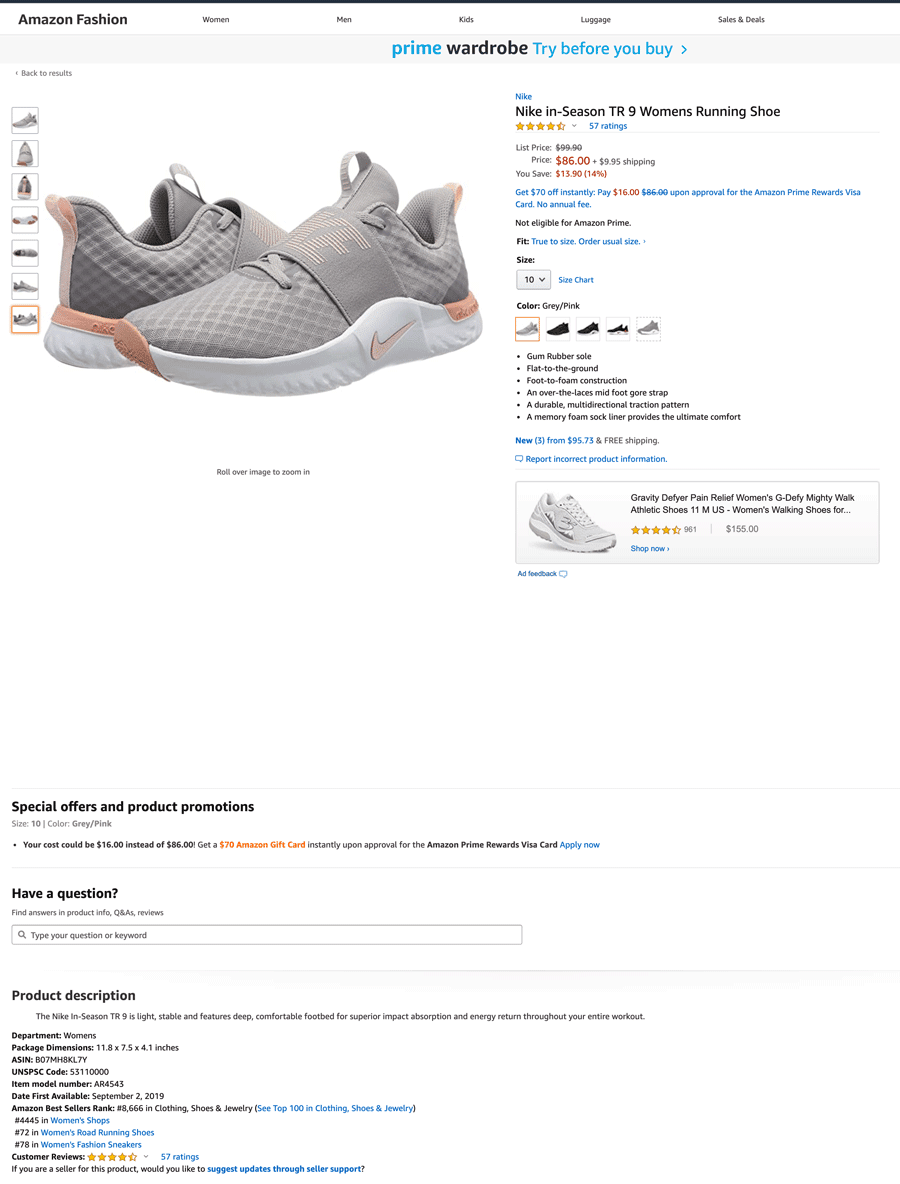Screenshot from Amazon Fashion showcasing the "Nike In Season TR9 Women's Running Shoe" priced at $86. The highly-rated shoes, nearly achieving a perfect 5-star rating from 60 reviews, are designed for lightweight comfort and style. Displayed in a gray color scheme, the shoes feature a peach accent on the top, under tread and swoosh, enhanced by a unique strap band for added support. White details complement the overall design. The product page offers eight clickable descriptions allowing customers to view the shoes from different angles and includes options to choose from five distinct color variations. A suggested alternative shoe appears with discount information and shipping details. Various sizes are available for order, and the zoom feature allows a closer inspection of the shoe's craftsmanship. A detailed product description is provided at the bottom of the page for comprehensive information.